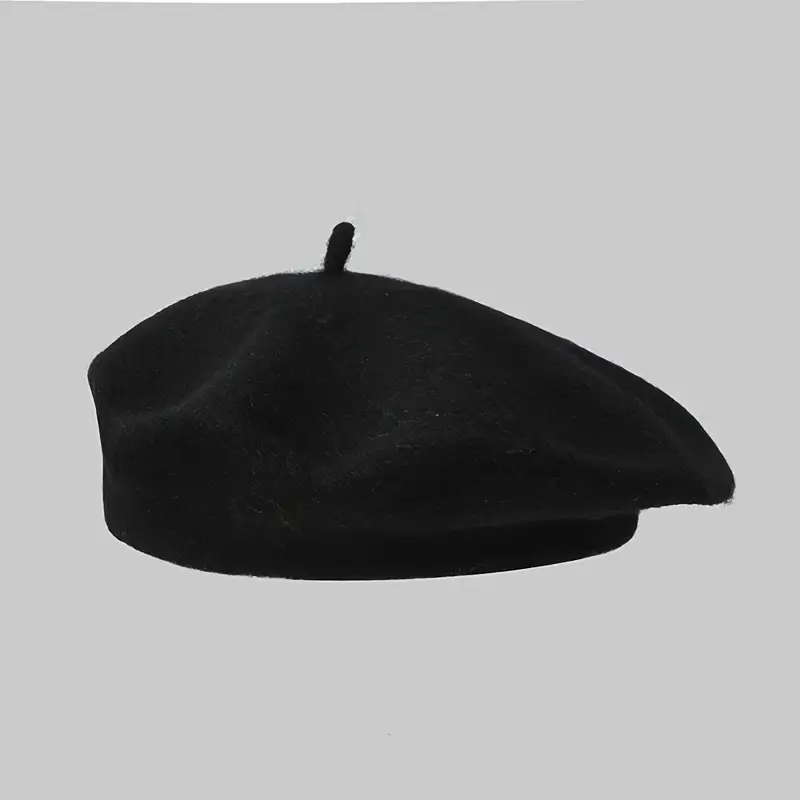The image showcases a black beret prominently positioned against a solid, textured gray backdrop. The beret, viewed from the side, highlights its distinctive characteristics: a round base with a part that flops over, and at the top, a small protruding strip of fabric. The material appears to be soft cloth, possibly felt, indicating some signs of use, as there seems to be lint on its surface. While the beret itself is the sole subject of the image, with no additional background elements, its placement and detailed capture suggest its potential significance, perhaps related to its age or former ownership.